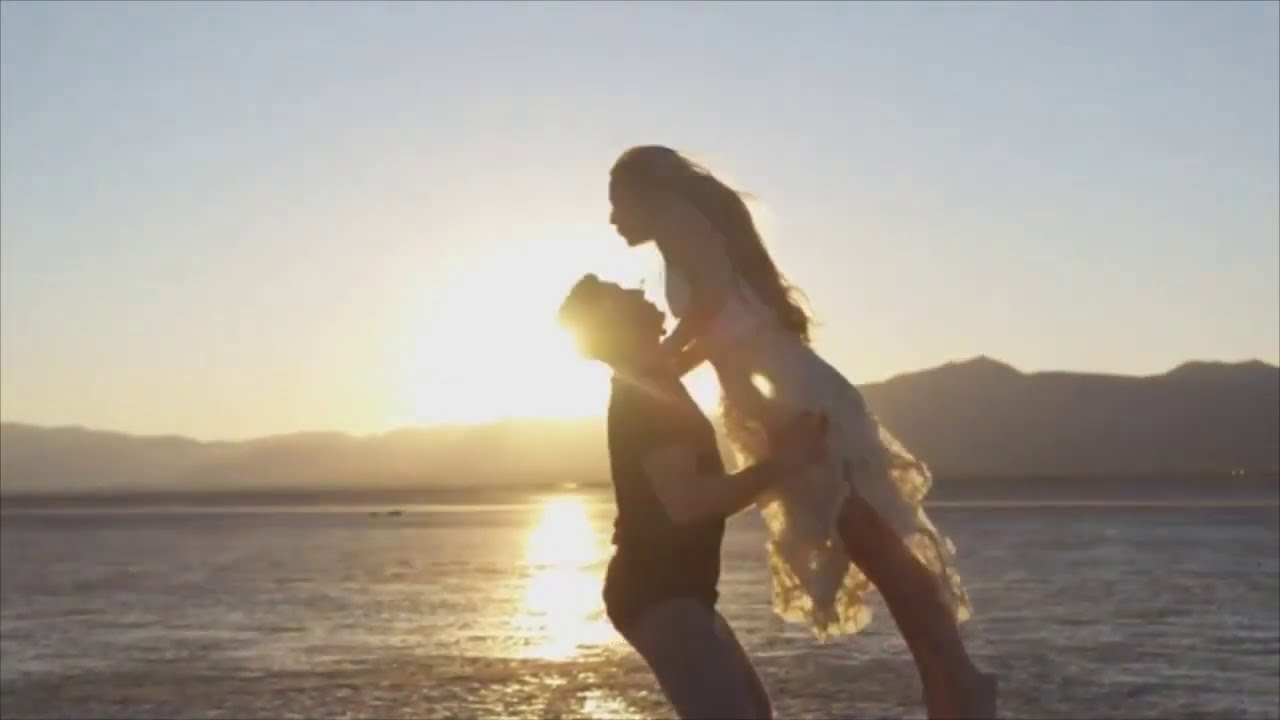In this captivating outdoor photograph, a man and a woman share a romantic moment against the breathtaking backdrop of a serene lake at sunset. The image, taken in landscape orientation, features the couple silhouetted by the soft, fading light of the sun as it dips behind distant mountains. The man, dressed in a black t-shirt and jeans, lifts the woman, who wears a light-colored, ruffled dress that falls to her calves. She leans into him, her hands resting on his shoulders and her long dark hair cascading down her back. The calm water of the lake reflects the warm, dusky colors of the sky, creating a tranquil and picturesque scene that highlights the couple's tender connection.